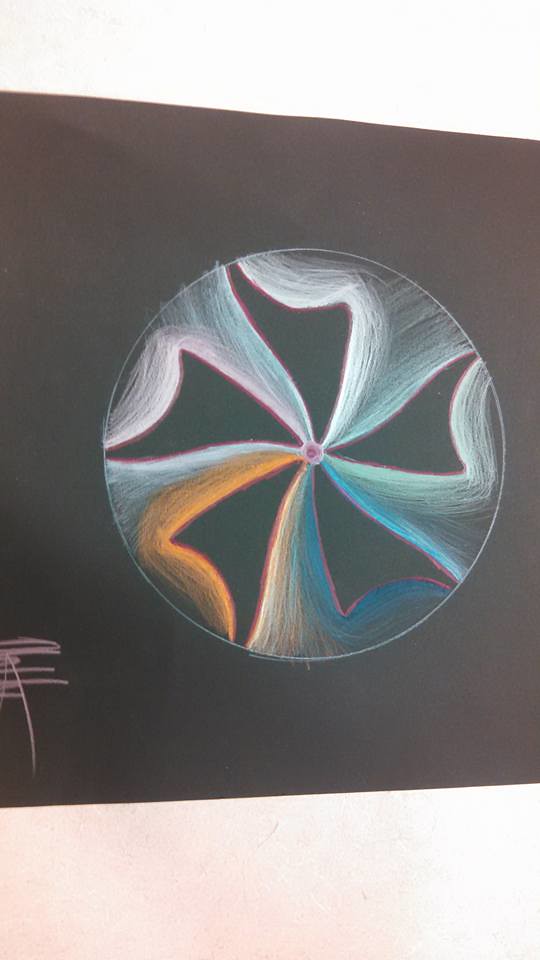An artistic drawing is showcased on black paper, meticulously hung against a beige wall. The photo captures the drawing, though the lower left-hand corner is slightly cropped out. The artist’s signature, characterized by a vivid pink scribble, is visible on the paper. The artwork, seemingly crafted with chalk, features a pinwheel design enclosed within a circle. This pinwheel comprises five blades artfully formed through the use of negative space, each outlined in striking red. The spaces between the blades are filled with a soft blue hue, adding depth to the composition.